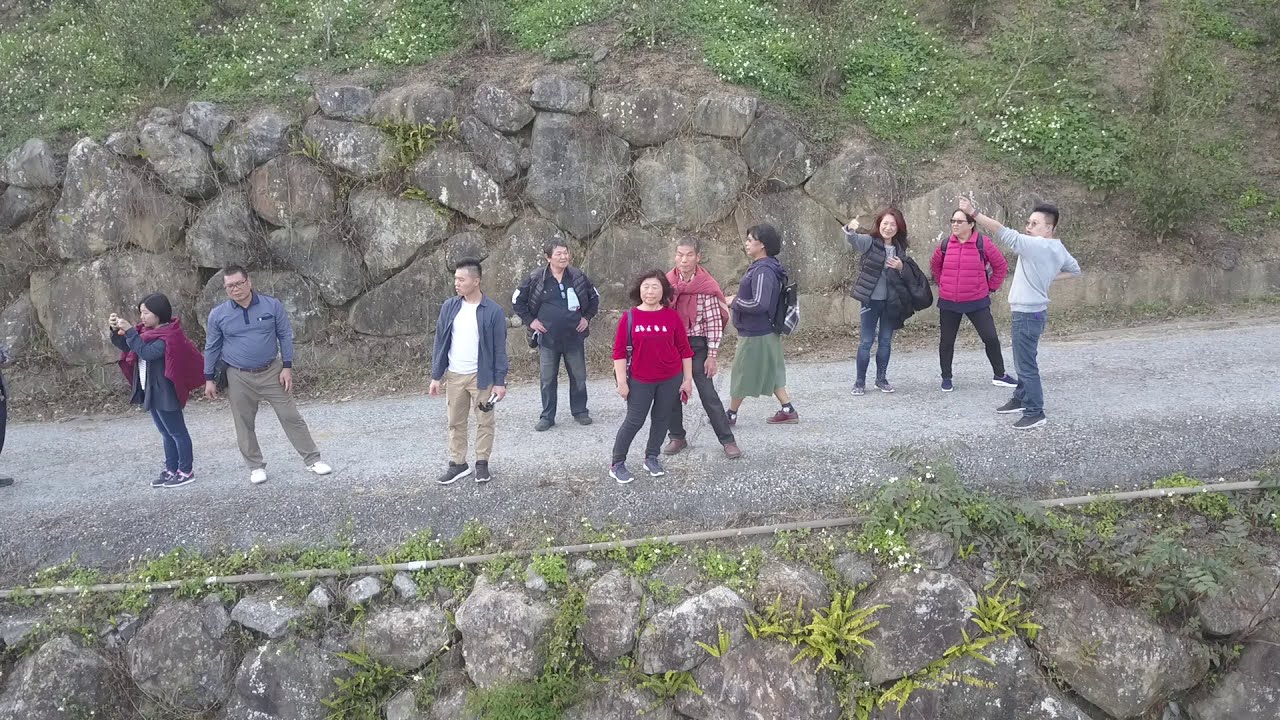This digital photograph captures a group of approximately 12 to 13 people of Asian descent standing and posing on a slightly tilted blacktop path that appears worn from foot traffic. The scene suggests an early fall season, as everyone is wearing coats in varying colors including red, black, blue, and tan. The pathway is flanked on both sides by rocky outcrops; the lower edge of the path is bordered by grayish rocks and greenery, while the higher edge features stacked rocks and more plant life, including small white flowers. The overall color palette of the image is diverse, featuring greens, grays, browns, and various clothing colors. Some members of the group are taking selfies, while others face the camera or look in different directions.